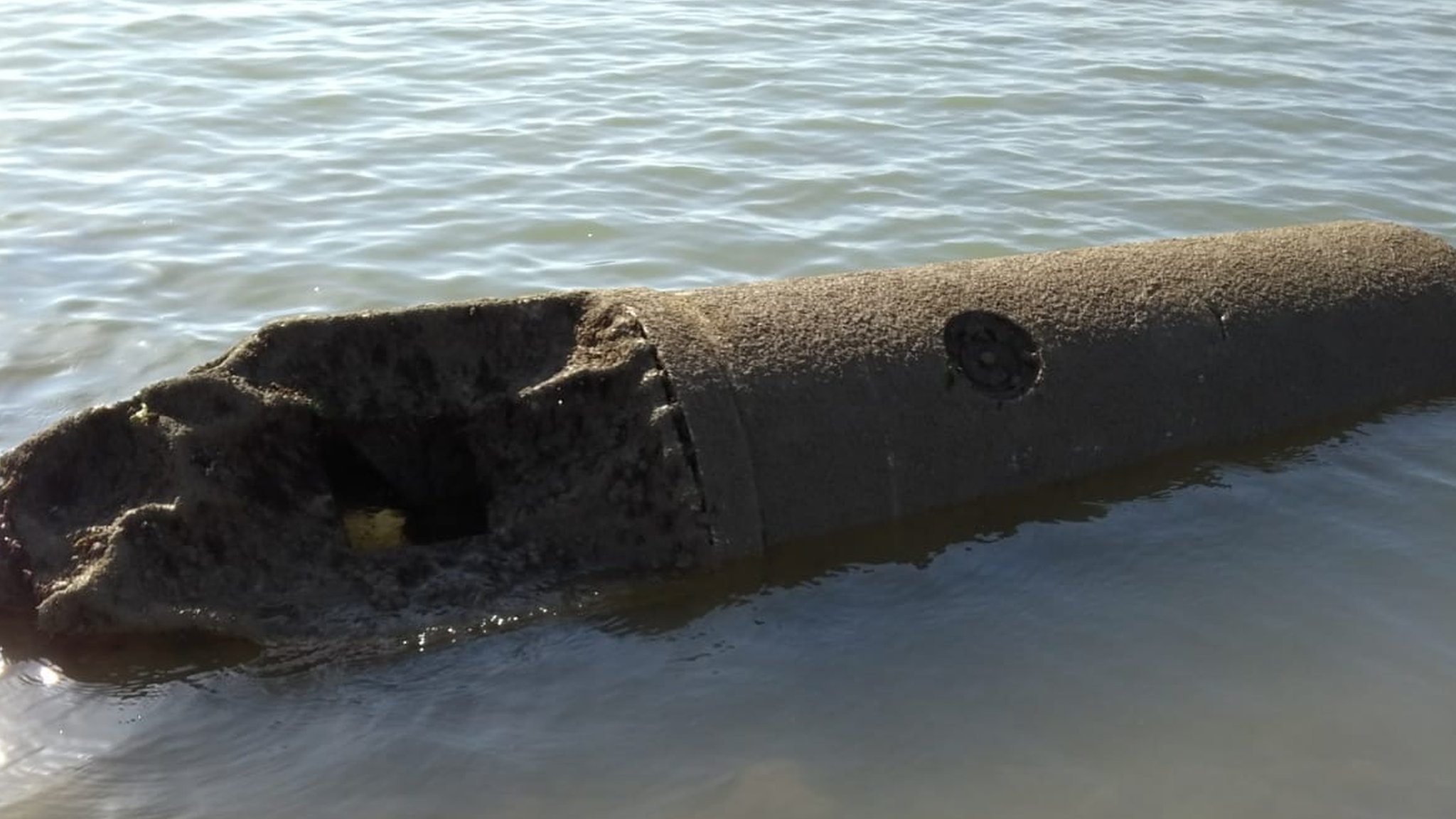This photograph depicts a heavily rusted and corroded World War II German sea mine that has washed up near Bognor Regis. The mine is cylindrical and long, reminiscent of a cigar shape, with a conspicuous circle at its center. The metallic surface is extensively decayed with visible bolts and nuts, and the front end appears to be missing or broken apart, revealing jagged edges and inner components. Despite being identified by some as a concrete structure, the predominant rusty metal features are apparent. The mine lies in a greenish-gray, stagnant pool of water, with little ripples stretching across the scene. This relic of war, haunting in its decay, contrasts starkly against the tranquil and slightly murky waters it rests in.